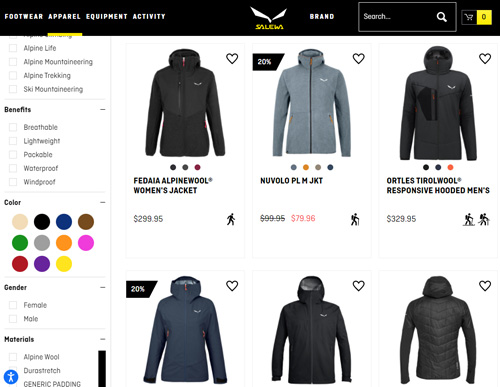The image shows an e-commerce website called "Salews," which specializes in footwear, apparel, equipment, and activities. Positioned in the upper left corner is the site’s logo featuring the name "Salews" spelled out clearly: S-A-L-E-W-S. The page being viewed focuses on winter and alpine jackets. 

In the upper right corner of the site, there is a search bar alongside an empty shopping cart icon highlighted with a yellow button indicating zero items. The left side of the page presents a scrolled-down menu displaying various categories and filters for jacket selection, including features like "Benefits" and "Materials." Under "Benefits," options such as "breathable" and "lightweight" are listed. Color options are available, allowing searches among 11 different colors: yellow, gray, green, blue, pink, orange, brown, cream, red, purple, and yellow. Gender filters are also provided for "male" and "female," and material choices include "alpine wool," "generic padding," and "DuraStretch."

On the main section to the right, six jacket options are visible. The first row shows three jackets with detailed pricing and information. These are a dark gray jacket, a light gray jacket, and another dark gray jacket. The second row features three more jackets, depicted in light and dark gray tones.

The first jacket listed is the "Fedea Alpine Wool Women's Jacket" priced at $299.95. The middle jacket is the "Povola PLM Jacket" with a price tag of $79.96. The last jacket is the "Ortelli's Tirola Wool Responsive Hooded Men's Jacket," costing $321.95. Each jacket has color dots underneath, indicating that they are available in multiple colors.